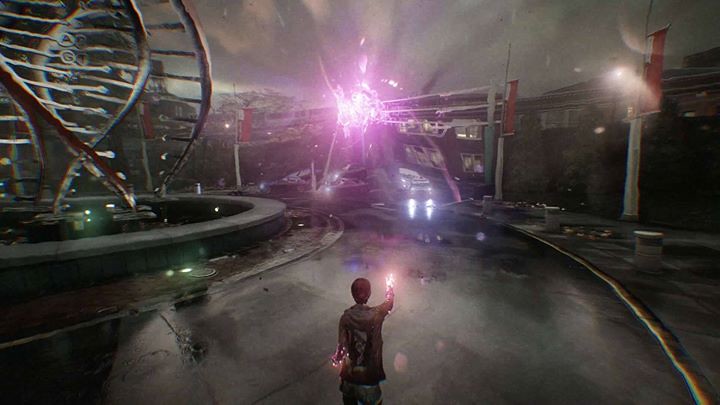This image is a screenshot from a sci-fi video game, evident from the computer-generated environments and characters. It features a 16x9 aspect ratio and depicts a modern-day setting with futuristic elements. The focal point is the player character, a young woman with short auburn hair, wearing a brown hooded jacket. Her hands are glowing a bright purple color, with the right hand pointed upwards and the left hand pointing downwards. In the top center of the image, a mysterious glowing purple light warps the scenery around it. The scene unfolds near a highway, complete with large signs and a bridge in the background. To the left, a metal sculpture resembling a DNA spiral with inscriptions "A" and "G" can be seen, accompanied by green lights, white or silver poles, and the shiny rain-soaked ground reflecting the ambient light.